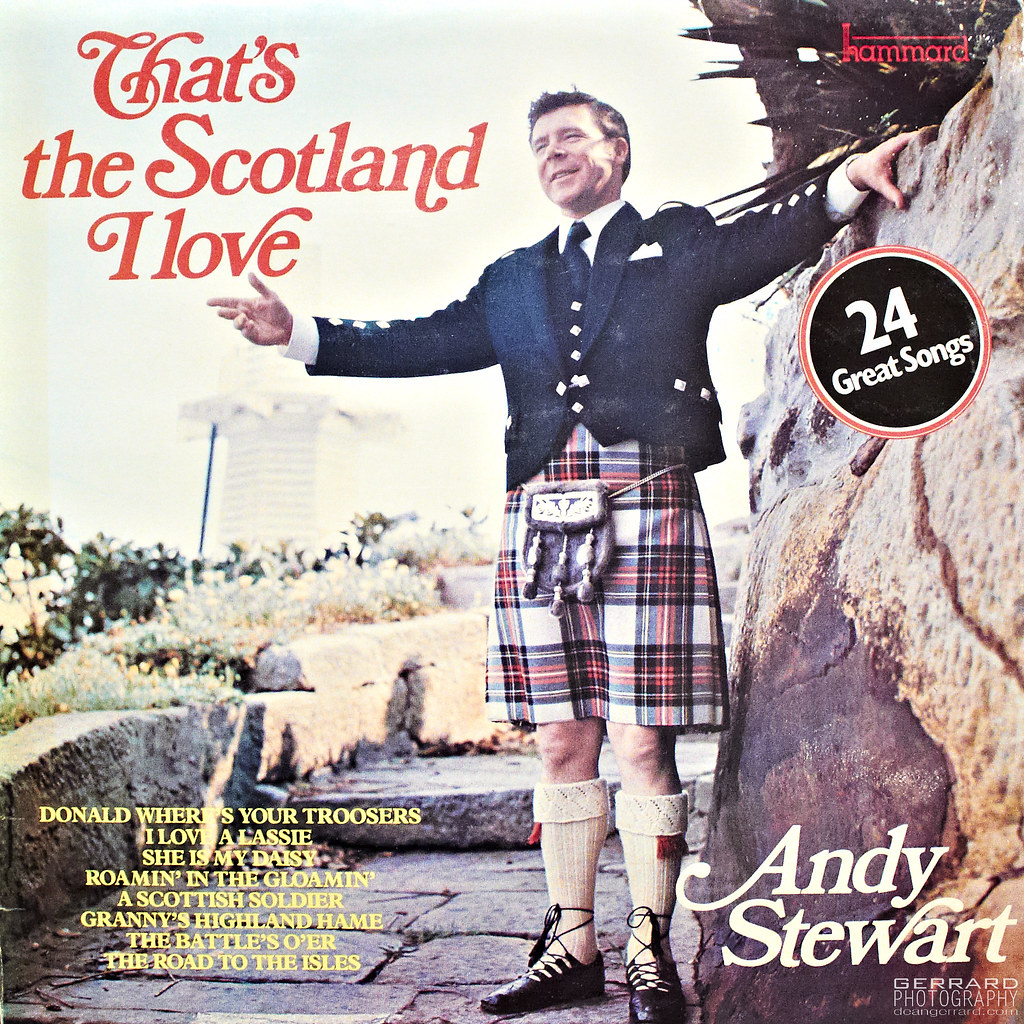The image appears to be a full-color promotional album cover. The square image features a man wearing a traditional Scottish kilt ensemble, comprising a plaid kilt, blue jacket, blue tie, and a handkerchief in his coat pocket. The man is positioned next to a large rock on a stone walkway, with his arms outstretched. The backdrop includes a tall white building, trees, bushes, and elements of a manicured garden. 

The text on the cover includes, in the upper left corner, "That's the Scotland I Love" in red text. In the upper right corner, also in red, it says "Hammered," spelled out as H-A-M-M-A-R-D. Below this is a black shaded circle with a white outline and white text that says "24 Great Songs." The lower right corner features the name Andy Stewart in white text, with the credit "Gerard Photography" just below it. In the lower left corner, yellow text lists several songs: "Donald Where's Your Trousers?," "I Love a Lassie," "She is My Daisy," "Roman in the Gloman," "A Scottish Soldier," "Granny's Highland Hame," "The Battles O'er," and "The Road to the Isles," along with the indication that there are a total of 24 songs.